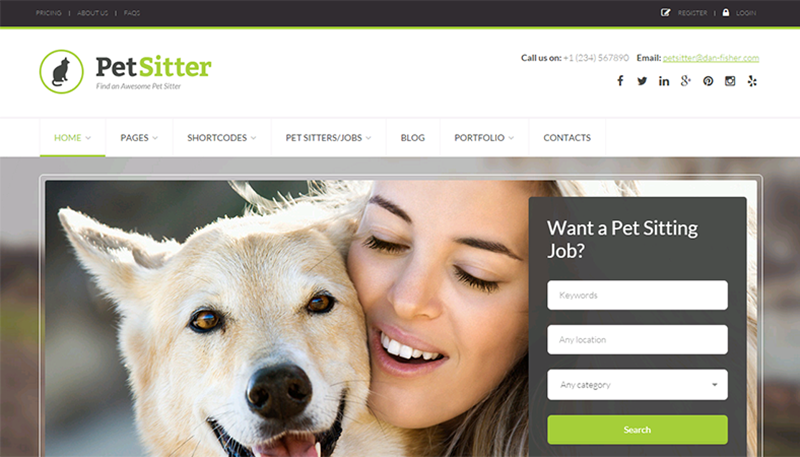This landscape-oriented screenshot of the PetSetter website features a sleek design with a black horizontal top border underlined in green. The top navigation bar is neatly organized, offering options in white text such as "Pricing," "About Us," and "FAQs." To the far right are "Register" and "Login" buttons framed in the same white font.

Beneath this, a prominent green circle with a white side showcases a black cat silhouette next to the site’s name, "PetSetter," where "Pet" is in bold black and "Setter" in vibrant green. Below this header, contact information including a phone number and email address is displayed, alongside an array of social media icons (Facebook, Twitter, Instagram, LinkedIn, Google+, Pinterest, and more).

The primary navigation tabs—"Home," "Pages," "Shortcodes," "PetSetter Jobs," "Blogs," "Portfolio," and "Contacts"—are aligned beneath the header, with the "Home" tab highlighted in green with a green underline. Below this, an engaging main image features a smiling blonde woman with bright white teeth, joyfully posing with her golden, wolf-like dog, both exuding happiness.

To the right of this dynamic duo, a gray vertical box catches the eye. It invites users to find "a pet sitting job" with white text, followed by input fields for keywords, location, and category. There is also a search bar, enabling visitors to look for pet sitting jobs effortlessly. This comprehensive screenshot effectively captures the user-friendly and welcoming essence of the PetSetter website.